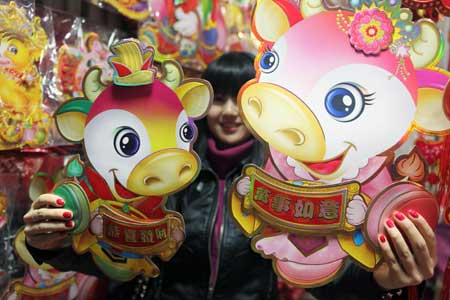In the vibrant, festival-like setting, an Asian woman with black hair, dressed in a green hat and jacket, stands as the focal point of the image. She holds up two large, cartoonish inflatable mascots, one in each hand, which resemble happy cows or pigs adorned with large yellow noses, big eyes, and wide grins showing pink tongues. The mascot on the viewer's left is red with a yellow hat, while the one on the viewer's right is pink with flowers in its hat. Both mascots sport an anime-style design and carry banners with Asian characters, further emphasizing the festive, possibly East Asian cultural theme. Background details include ornate and brightly-colored decorations typical of fairs or festivals, adding to the celebratory atmosphere of the scene.